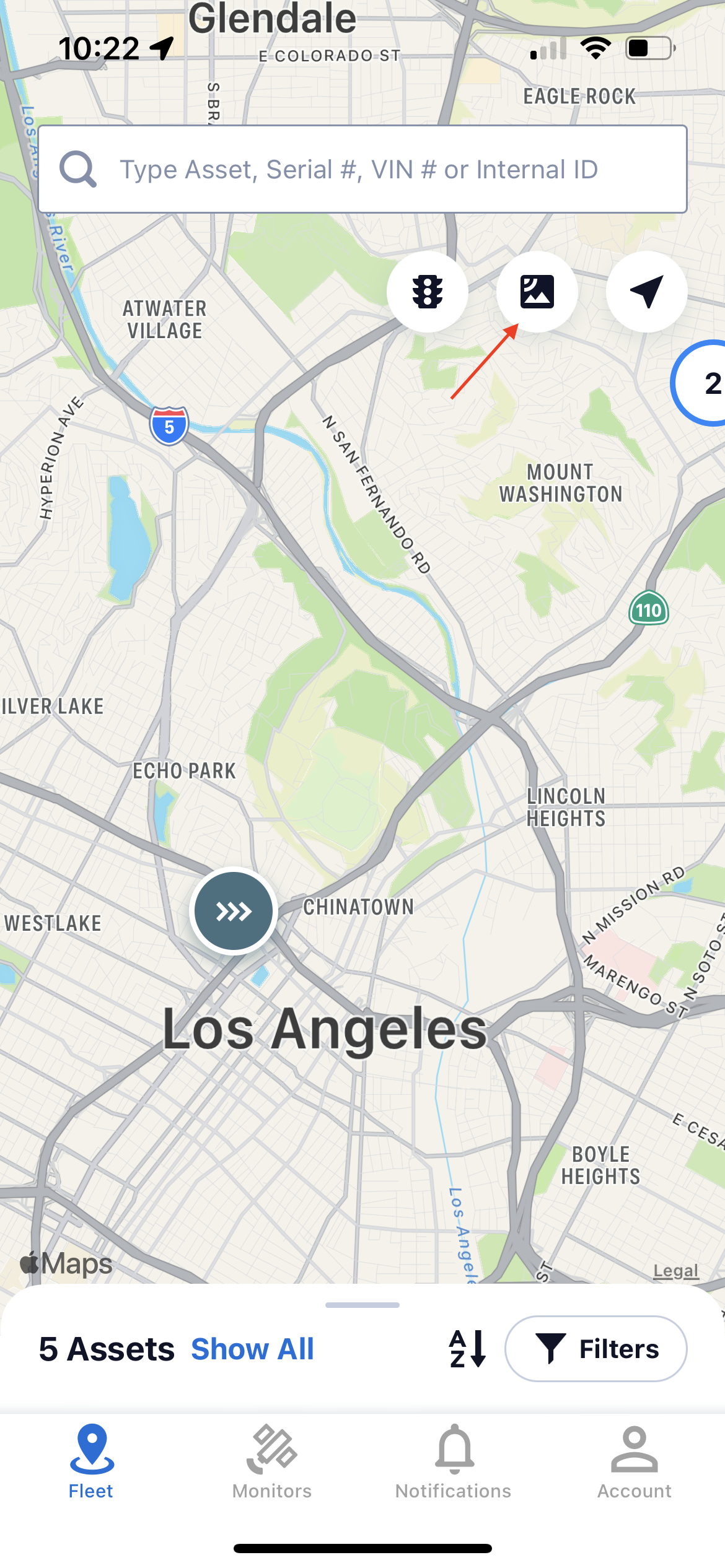This image appears to be a screen capture of a navigation or transportation app interface, displaying a map of the Los Angeles area. 

In the top left corner, the number "1022" is visible alongside the GPS icon. On the right side of the screen, the status bar shows a single bar of cell signal, a full Wi-Fi signal, and approximately 50% battery remaining, as indicated by the battery icon.

The map itself is predominantly gray, with darker gray lines representing major highways and interstates. Some of the roads are marked in white, black, and darker black lines. Notable labels include "Glendale" near the top left-center and "Los Angeles" about three-quarters down to the bottom left-center. Just above the "Los Angeles" label, there is a white circle with a green interior containing three arrows pointing to the right.

Key landmarks and areas identified on the map include I-5, Highway 110, Chinatown, Echo Park, Lincoln Heights, Bowling Heights, and Westlake. Some of the specifically marked roads are East Colorado Street and North Mission Road, although other road names are not legible.

At the bottom of the image, there are several functional sections. In black text, the notation "5S" appears with a blue "Show All" button. Below these, a blue button labeled "Fleet" is present. Additional sections in gray text include "Monitors," "Notifications," and "Account."

This detailed navigation or transport app screenshot offers a comprehensive view of the Los Angeles area, highlighting major roads, neighborhoods, and interface elements.